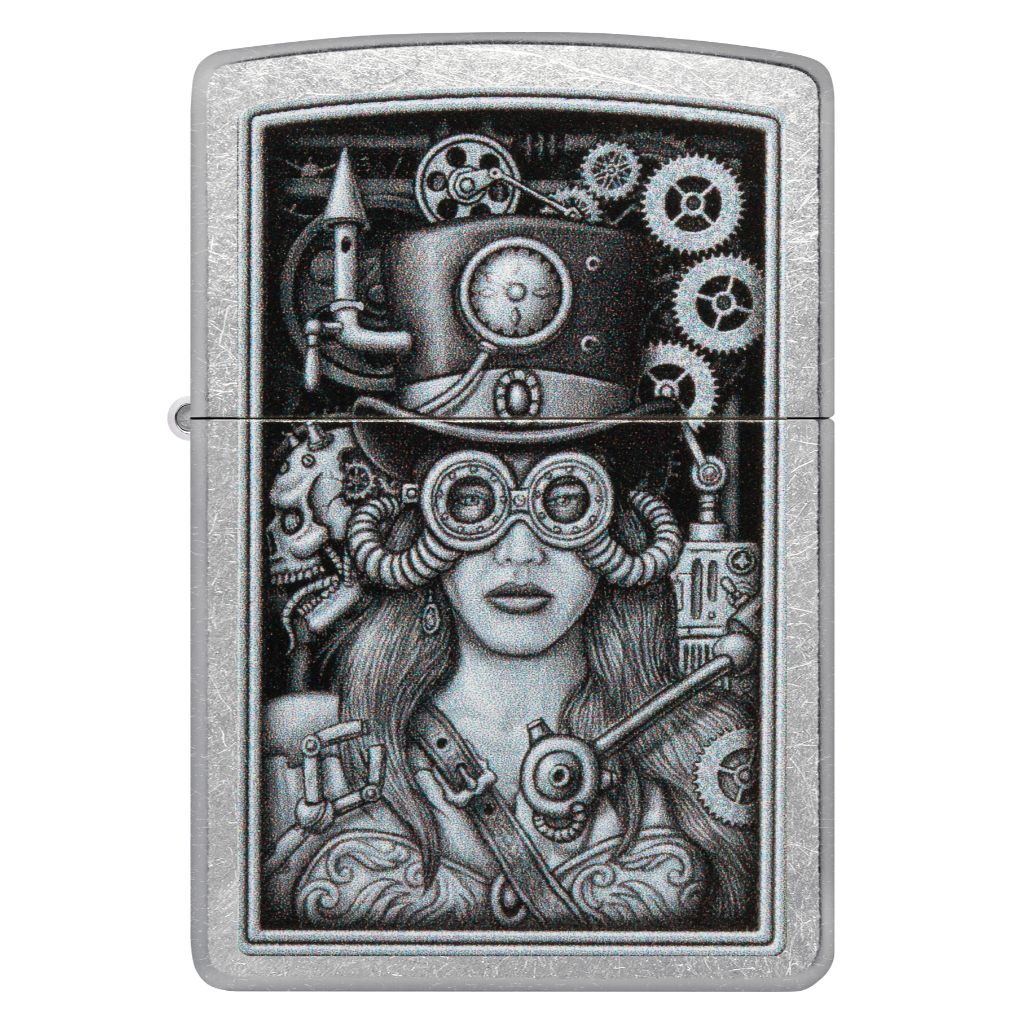This is a close-up photograph of an ornately designed lighter, showcasing a detailed and somewhat distressed metallic exterior. The front-facing design is etched in black, white, and gray tones, displaying an intricately crafted steampunk scene. Central to the artwork is a steampunk woman with shoulder-length hair, adorned in a metal brassiere and a top hat fitted with a pressure gauge and steam whistle. She wears goggles with tubes wrapped around her head, linking her to a complex backdrop of gears and machinery. To her left, a skull embellished with cogs and metal components adds to the industrial, cyberpunk aesthetic. The whole composition exudes a rough, distressed charm, blending Victorian and futuristic elements seamlessly.